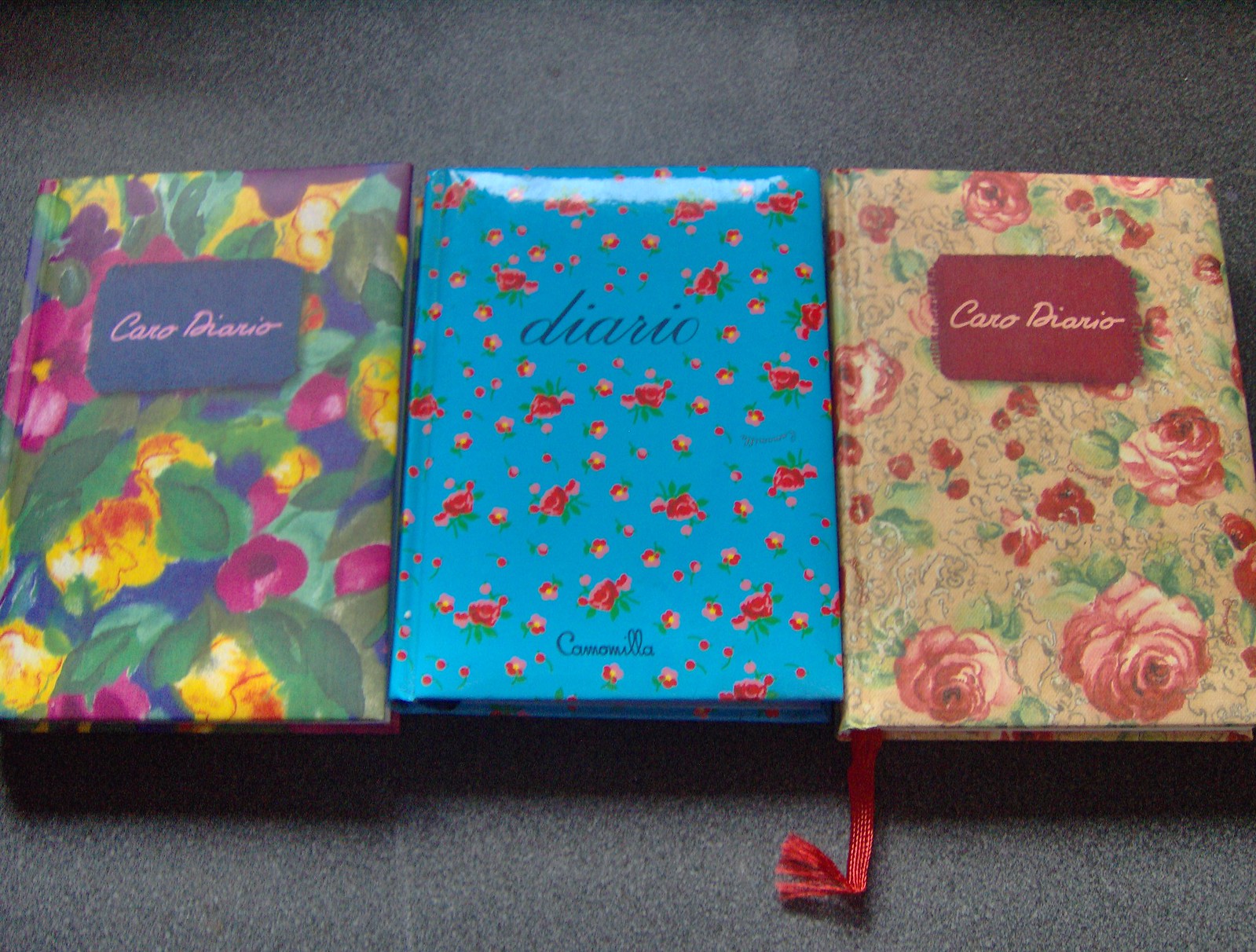The image features three elaborately designed diaries laid side-by-side on a black and grey speckled surface that appears to be either an epoxy countertop or flooring. Each diary showcases a different floral pattern, with the covers designed in vibrant colors and detailed illustrations. 

The diary on the far left displays a motif of green leaves with purple and yellow flowers, centered with pink text in a black box that reads "CARO DIARIO." The middle diary is a baby blue color adorned with smaller, more sparsely arranged red roses and green leaves. It has black text at the top that says "DIARIO" and at the bottom, "CAMOMILLA." The diary on the far right has a beige or tan background with large pink and red cabbage roses and green leaves. It also features a prominent red box with the text "CARO DIARIO" and includes a red tassel bookmark hanging from the bottom.

All three diaries are aligned in a row on the speckled surface, their colorful and artistic designs made even more striking by the close-up perspective of the image.